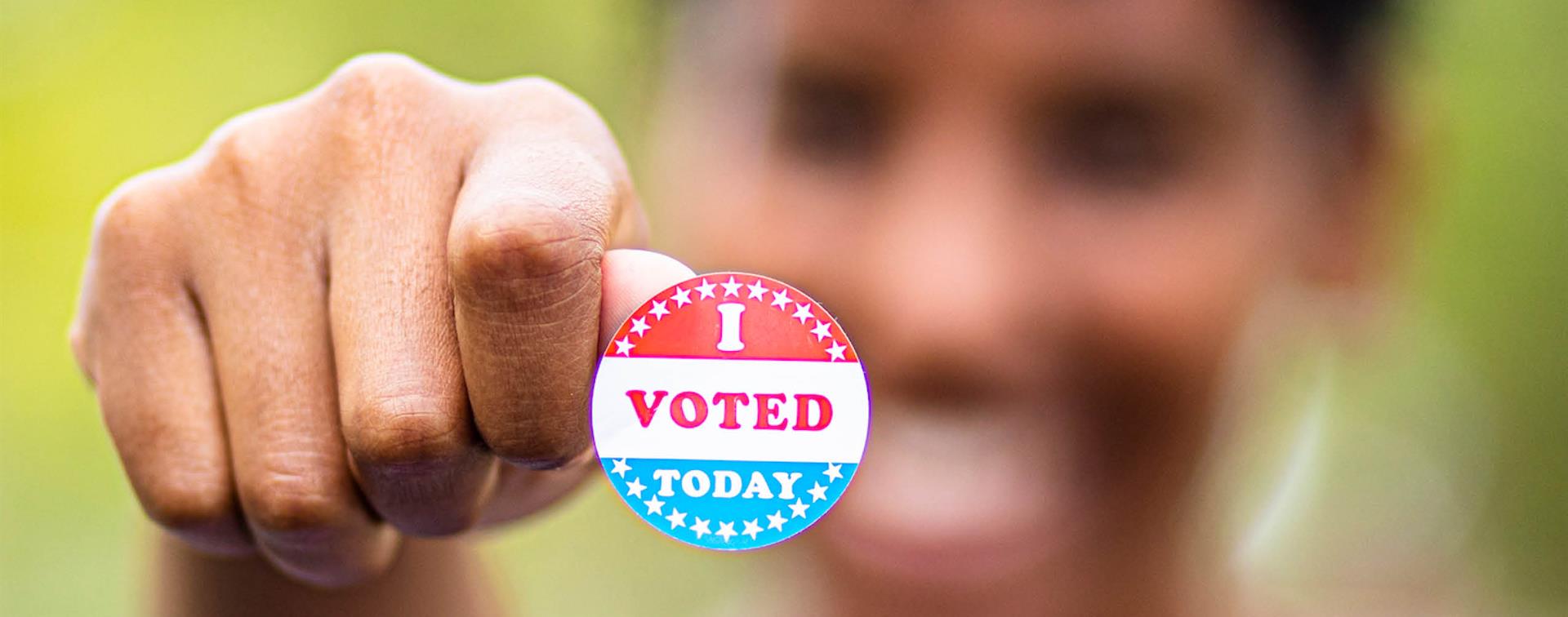In the foreground of this image, a clear right hand, likely of a young Black woman, displays a circular "I Voted Today" sticker on her thumb. The sticker features distinct sections: a red top with white stars and the letter "I," a white horizontal banner in the middle with "VOTED" in bold red capital letters, and a light blue bottom with white stars and "TODAY" in capital letters. The backdrop is blurred, portraying green foliage, possibly a forest. Although the person in the background appears to be smiling, the details are too indistinct to confirm facial features or expressions accurately.